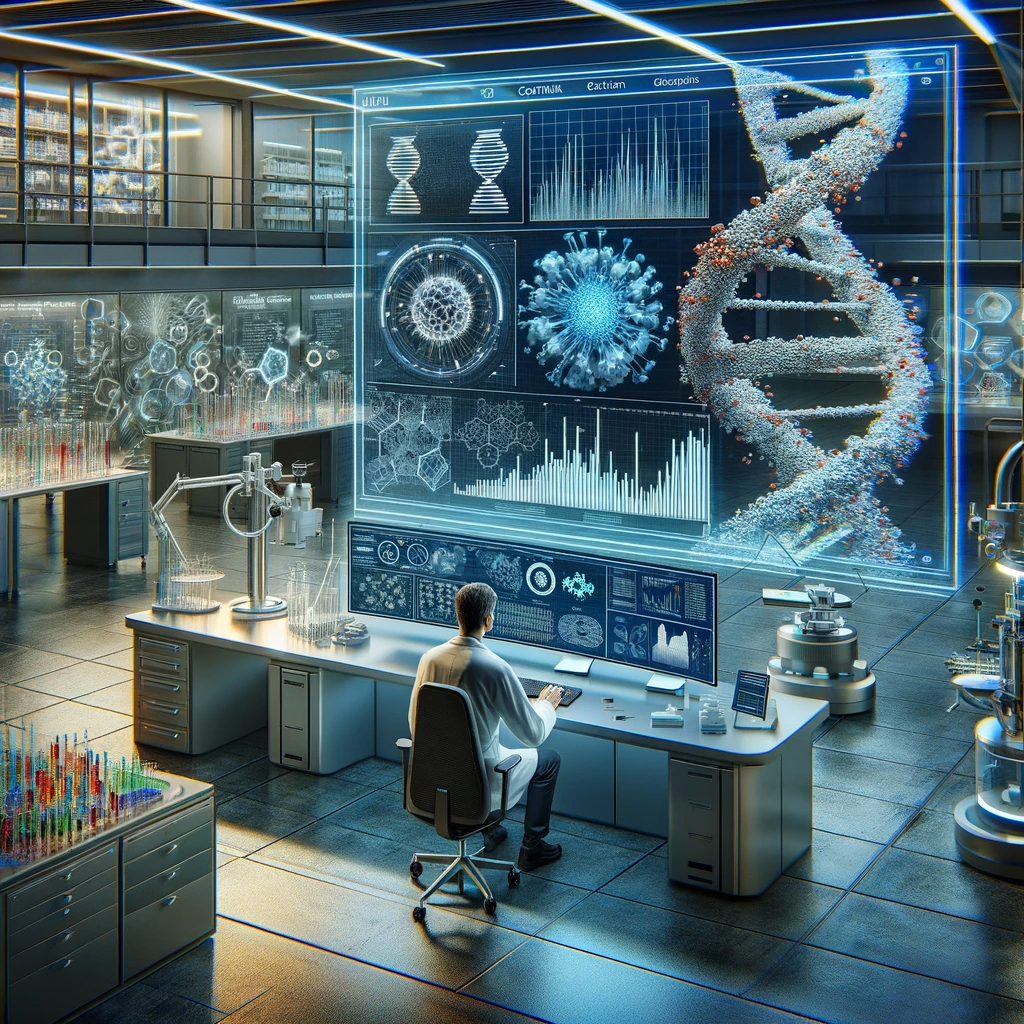This intricate color illustration depicts a bustling high-tech laboratory environment. Dominating the scene is an expansive computer monitor filled with multiple complex diagrams. Positioned at the right edge of the screen is a detailed model of a white DNA strand, signifying the scientific nature of the work. In the foreground, a long white desk is strewn with various scientific apparatus, including microscopes and test tubes, suggesting active experimentation.

Seated at this desk is a researcher, identifiable by their white lab coat and dark pants. They are engaged with another set of computer terminals, typing away on a keyboard. A closer inspection reveals the AI-generated nature of this image, evident from the uncanny appearance of the person’s hand.

To the image’s left, a walkway leads to rooms with large glass windows, behind which more scientific equipment can be observed, indicating a well-equipped and comprehensive research facility. Flanking both sides of the image are numerous tall, multicolored test tubes, adding a vibrant and dynamic visual element.

The laboratory's pristine interior is emphasized by the bright, tiled white floor, contributing to the overall sense of cleanliness and precision in this advanced scientific setting.